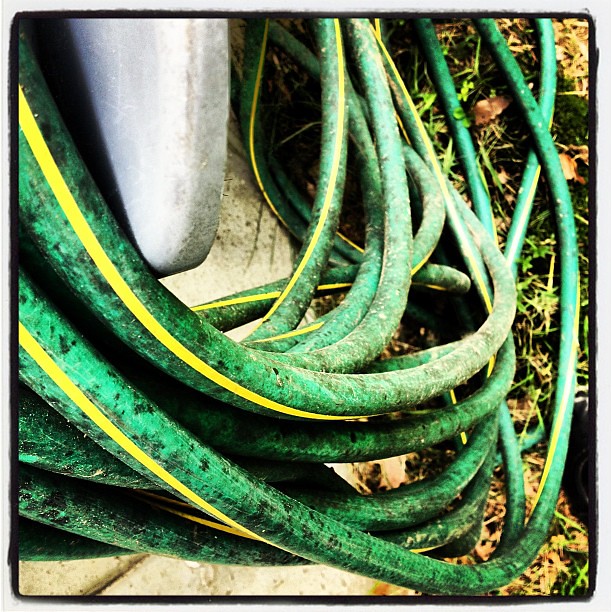The photograph captures an outdoor scene featuring a green garden hose with a yellow stripe running its length. The hose appears noticeably dirty, covered in a layer of dust and dirt, and is partially coiled around a structure in a somewhat haphazard manner—with part of it neatly wound and the rest piled messily on the ground. This green hose with a yellow accent lies atop both a partially grassy area, which includes patches of brown and green grass. The grass is scattered and slightly sparse in some areas, revealing glimpses of dirt beneath. In the bottom left corner, concrete pavers or tiles are visible, edging into the grassy area. The upper left of the image shows a silver oval-shaped object and a suggestion of a structure, possibly resembling a blue bicycle seat or a white stone wall, although details on these are less clear and somewhat obscured by dirt. There are a few brown leaves dotted across the scene. The overall image is framed with a small black border, set against a white background.